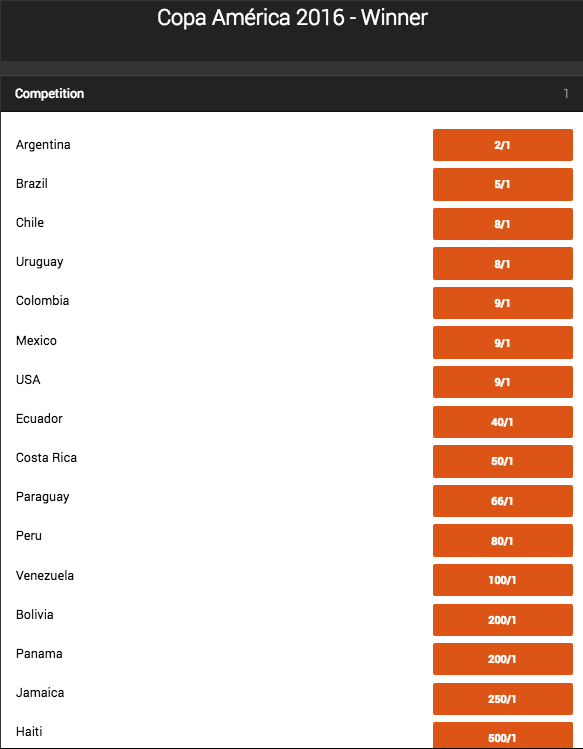This image is a narrow screenshot, likely taken from a smartphone, featuring content from a detailed sports summary. The background is predominantly white with a dark gray section at the top displaying the headline in white text: "COPA América 2016 - Winner." The word "América" includes an accent mark, reflecting its Spanish spelling. 

Below the headline, the word "competition" is positioned on the left side against the white backdrop. The left side of the image lists the participating countries in a vertical format. The right side features a corresponding column of orange rectangles, each containing white numbers to represent the results or rankings of the countries listed. 

From top to bottom, the countries listed are:

1. Argentina
2. Brazil
3. Chile
4. Uruguay
5. Colombia
6. Mexico
7. USA
8. Ecuador
9. Costa Rica
10. Paraguay
11. Peru
12. Venezuela
13. Bolivia
14. Jamaica
15. Haiti